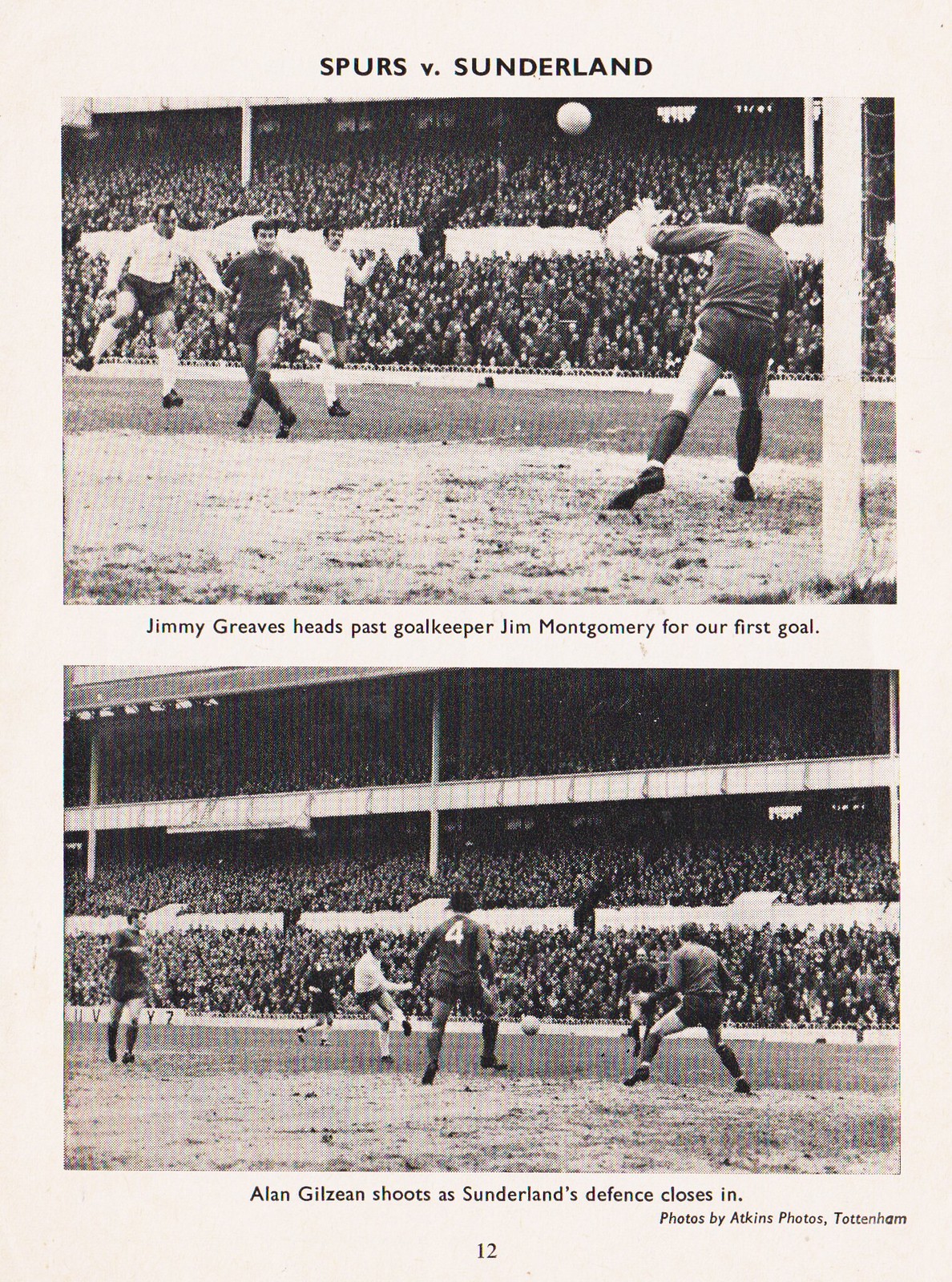The page, with an off-white cream background, resembles an old sports magazine and showcases two black-and-white photographs of a historic soccer match, Spurs versus Sunderland. At the top, the title "Spurs vs. Sunderland" precedes the first image, which captures a tense moment on the field. In this evocative scene, goalkeeper Jim Montgomery, arms and legs outstretched, prepares to block a ball as three players, two in white shirts and one in a darker shirt, vie for the ball. The packed stands in the background indicate a full-house witness to this gripping encounter. The caption below reveals, "Jimmy Greaves heads past goalkeeper Jim Montgomery for our first goal." The second photograph, situated below, displays another intense interaction with players surrounded around the ball on what appears to be a slightly rough, dirt field. One player, with the number four visible on his back, is prominently featured. Again, the stands are filled with attentive spectators. The accompanying caption reads, "Allen Gilzean shoots as Sunderland's defense closes in." At the very bottom of the page, the photo credits state "Photos by Atkins Photos, Tottenham," and the number 12 is displayed centrally.